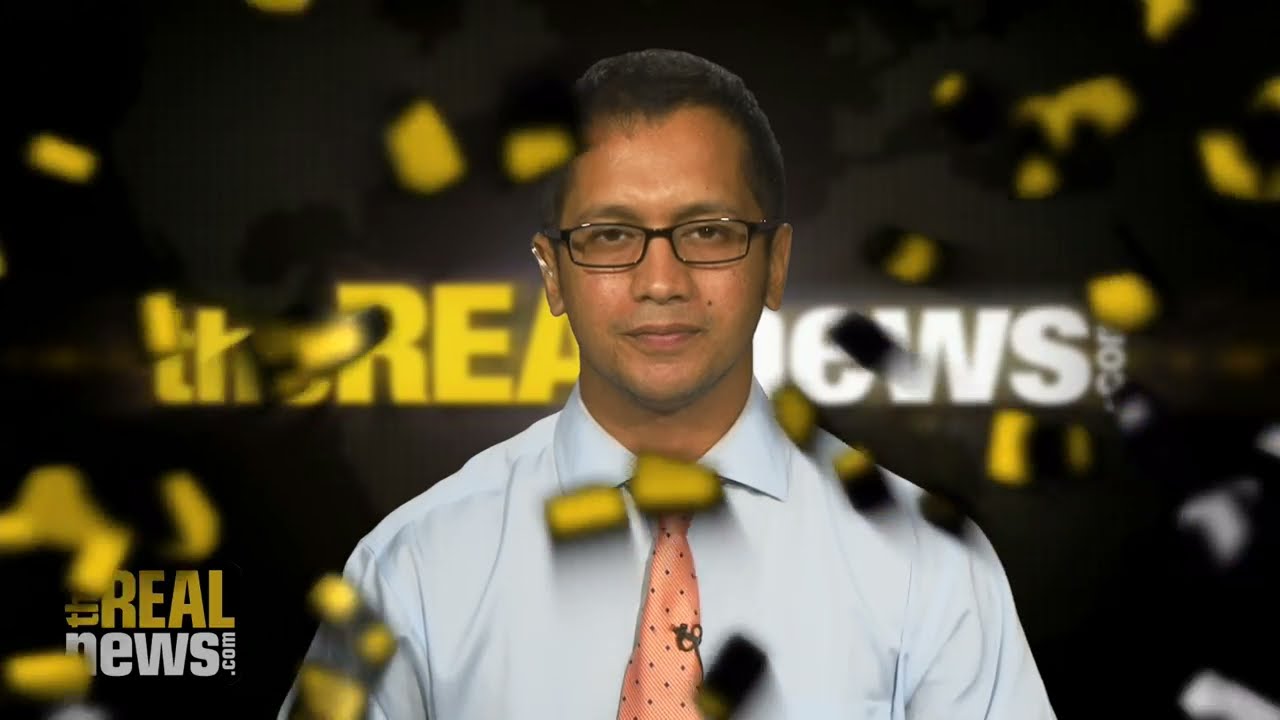In the center of the image, there's a man who appears to be of Indian or Hispanic descent, characterized by his dark eyes, dark short hair, and a distinct mole on his right cheek near his nose and mouth. He wears rectangular black-framed glasses and is dressed in a light blue or white button-down shirt paired with a salmon or peach-colored tie adorned with polka dots. A pen or microphone is clipped to his tie. His facial expression is nonchalant, with a slight smile that doesn’t reveal his teeth. Additionally, he has a white earpiece in his right ear, suggesting he might be receiving instructions.

The background is predominantly black but features understated yellow and white elements along with the website "therealnews.com" prominently displayed twice in yellow and white lettering. In the lower left corner of the image, the website is mentioned again in white. Yellow and black confetti are scattered around the man, adding a celebratory or dynamic feel to the scene. The overall impression is that the man is a broadcaster or presenter for "therealnews.com," highlighted as the focal point against this visually engaging backdrop.